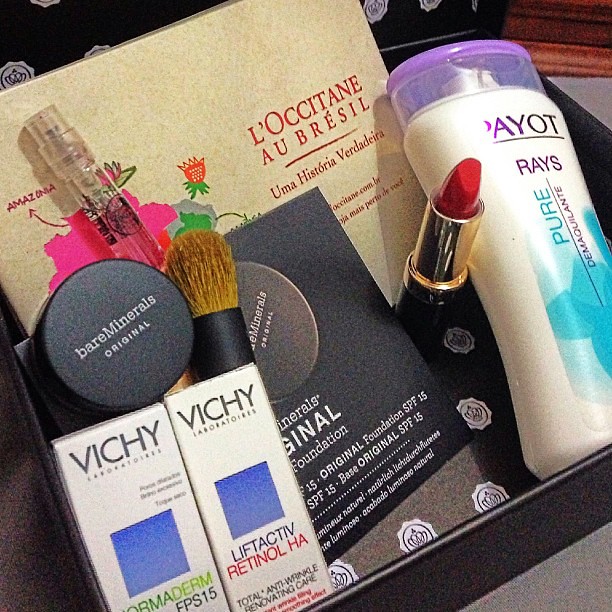The image depicts an open black gift box lined with black paper featuring a logo of a circle surrounding a crown. Inside the box, there is an assortment of beauty and skincare products. Dominating the scene is a bright red lipstick prominently displayed. To the right of the lipstick is a white bottle with a purple top labeled "Payot Rays and Pure". Behind these items is a beige pamphlet with pink and red lettering, indicating it's from L'Occitane au Brésil. Adjacent to these is a black compact labeled "Bare Minerals Original" in white writing, accompanied by a cosmetic brush. In the lower left-hand corner of the box, there are two white boxes with blue squares in the middle, branded "Vichy," one of which specifies "Retinol HA". Additionally, there is a clear white glass bottle, likely a perfume sample, and a black card tucked behind the other items.